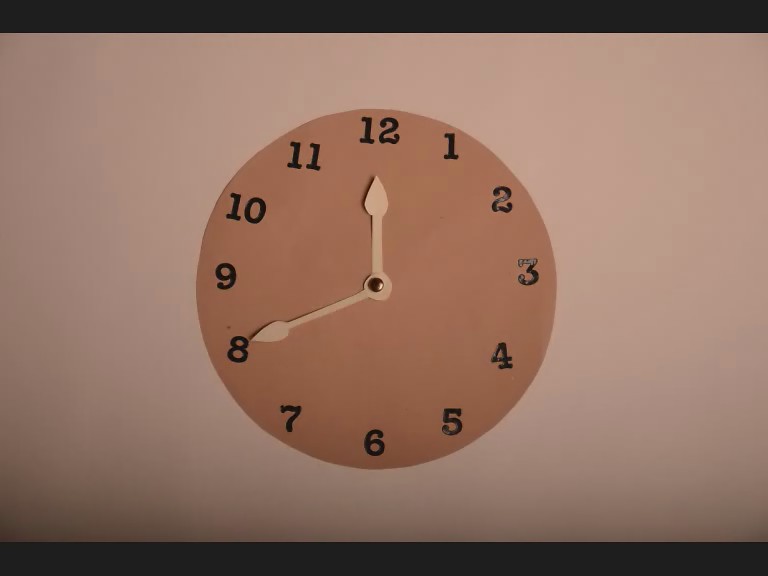The image showcases a hand-drawn clock face on a white sheet of paper, likely part of a child's art project or educational tool. The clock has a slightly irregular brown circular face, emphasizing its freehand origin. Black numbers from 1 to 12 are meticulously drawn around the clock's perimeter. In the center, a gold-colored pushpin-like button secures the clock's hands, which are a beige or manila color, each ending in spade-like points. The overall image has a horizontal orientation and displays noticeable shadows, particularly in the bottom left corner, giving it an unprofessional and homemade appearance against a plain white backdrop.